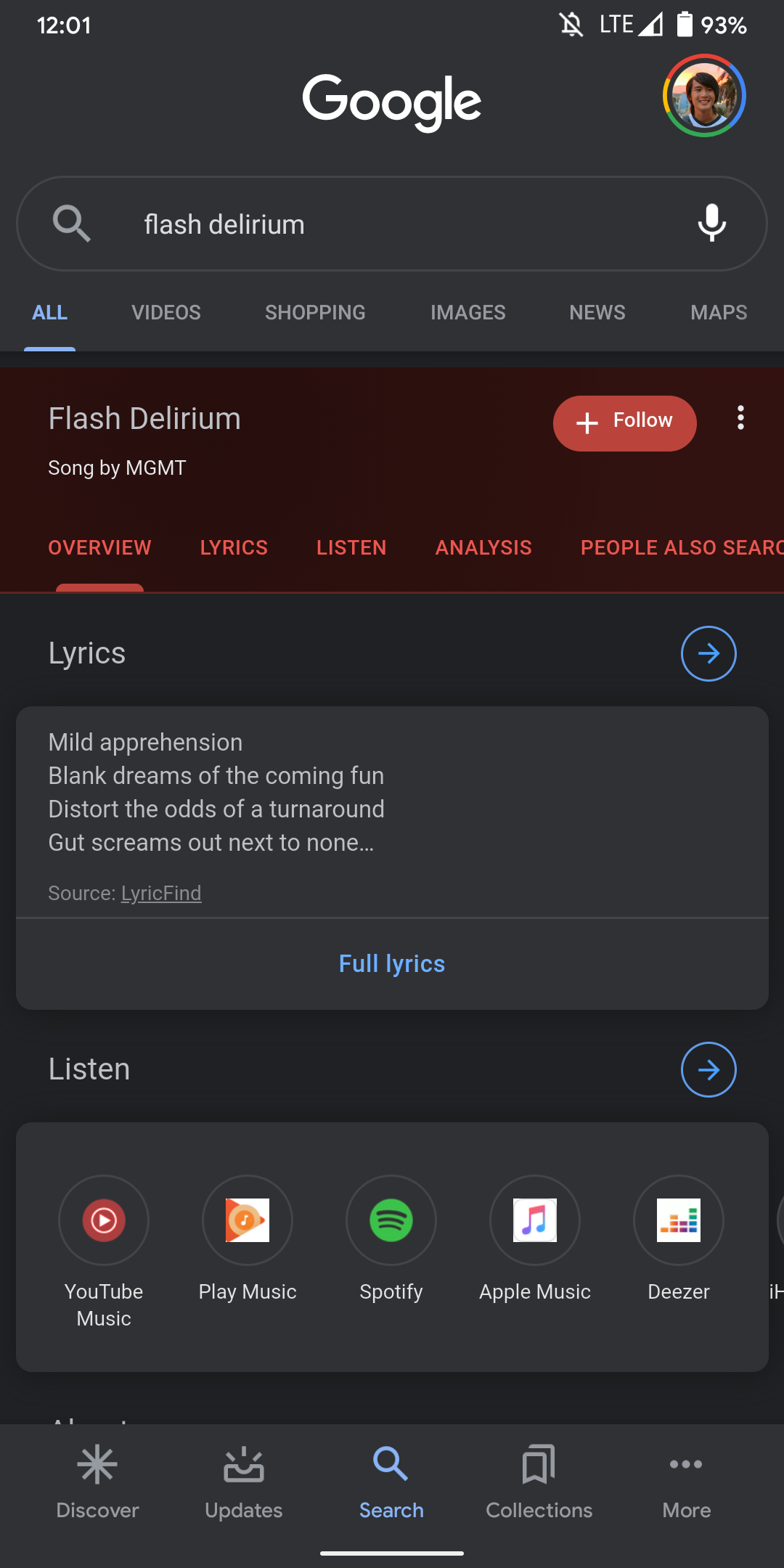The screenshot showcases a cellular phone interface with a vertical image orientation, approximately two and a half to three times taller than its width. The background is predominantly gray. In the upper left corner of the screen, white text displays the time as "12:01." The top right corner includes various status icons: an alarm off signal, LTE connectivity with full signal strength, and a battery icon indicating 93% charge.

Prominently centered in white text, "Google" is displayed beneath the status bar. Adjacent to it on the right is a small profile picture. A search bar occupies the next section, showcasing the user's recent search query "Flash Delirium" in white text. Below the search bar, Google’s navigation tabs include options like All, Videos, Shopping, Images, News, and Maps. The "All" tab is selected, highlighted in light blue with an underline, while the remaining tabs are gray.

The content area transitions into a dark red background for about 20% of the display height. On the left side within this section, "Flash Delirium" is prominently shown in white text, and is identified as "Song by MGMT." To the right, a follow button is displayed, labeled "Follow" in white text with a plus symbol on the left.

Below this, a lighter red section introduces another navigation menu featuring categories such as "Overview," though details beyond this brief appearance are not fully visible within the screenshot.